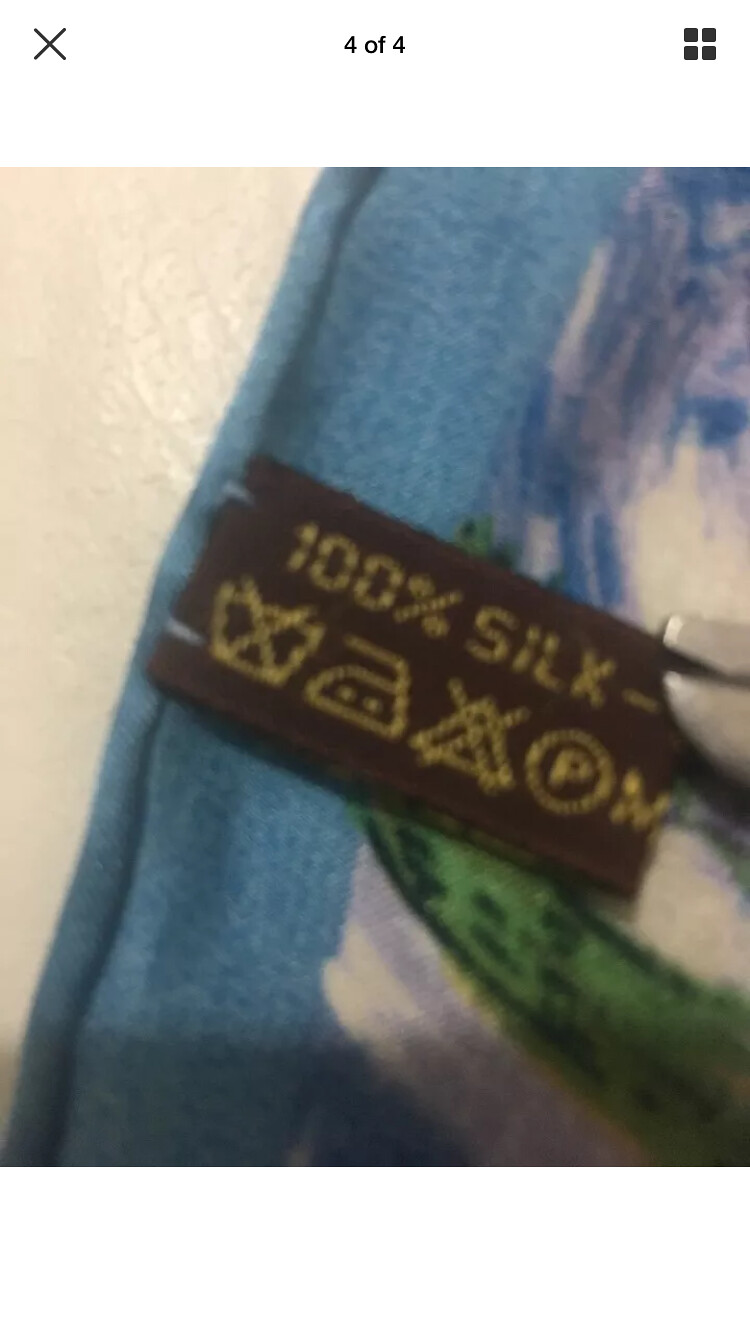This extremely close-up photograph captures a brown tag on a piece of blue fabric, likely an item of clothing. The tag features yellow text that reads "100% silk," and below it, various symbols provide care instructions on washing, ironing, drying, and dry cleaning. On the right side of the image, intricate stitching—possibly an artwork or design—is visible on the blue fabric. Interestingly, the image appears to be a screenshot from a photo app, indicated by a top bar displaying a white space with a "404" in the center, an X icon in the top left, and a 2x2 grid of squares in the top right.